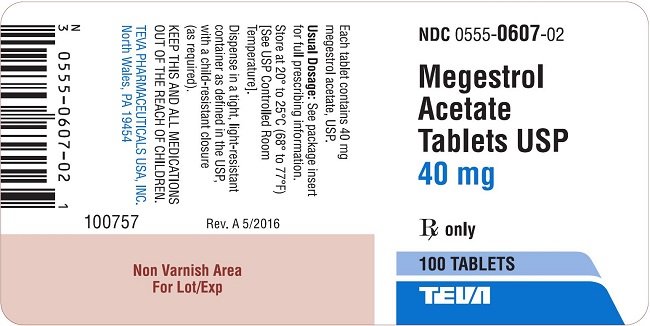The image displays a pharmaceutical label for Megestrol Acetate Tablets USP. On the right-hand side of the label, "Megestrol Acetate Tablets, USP" is prominently printed in black, alongside "40 mg" in blue. Below this, the label specifies "RX only" followed by "100 Tablets." The manufacturer's name, presumably "TEVN," is also indicated. At the top right section, an NDC number, "0555-0607-02," is displayed for reference.

On the left-hand side, a pink bar with red lettering states, "Non-varnish area for lot/expiration." Above this bar, detailed usage information is provided: "Each tablet contains 40 mg Megestrol Acetate USP. Usual dosage: See package insert for full prescribing information. Store at 20°C to 25°C (68°F to 77°F)." Additionally, the label advises to "Dispense in a tight, light-resistant container as defined in the USP."

The label's overall design ensures that all critical information for the safe and proper use of the medication is clearly presented.